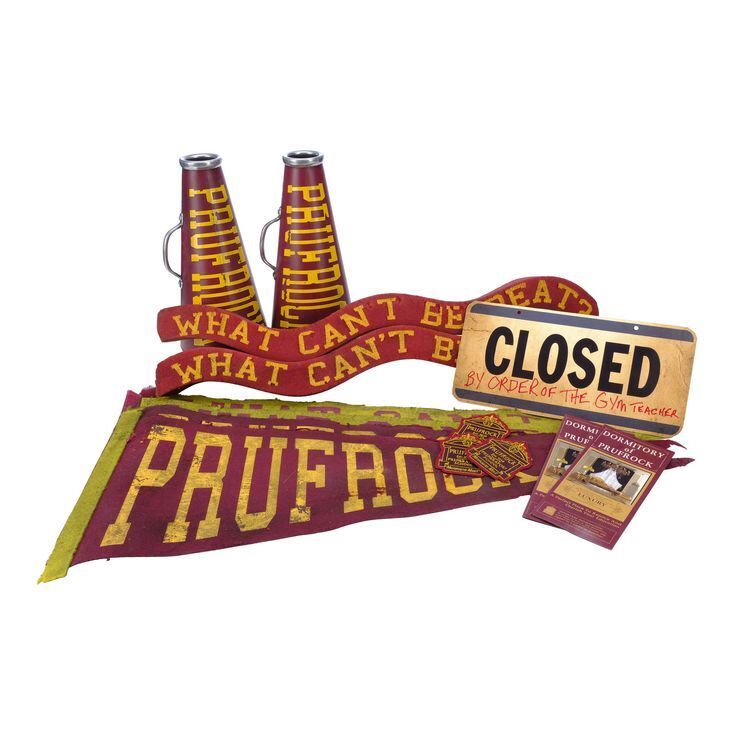The image depicts various items arranged against a white background with no border. Dominating the top portion are two comb-shaped speakers or megaphone-like objects in dark brown or red hues, each with a metallic handle and tip. Written vertically on these objects in yellow letters is the word "PRUFROCK," extending from the narrow top to the wider bottom. Below them, two curved banners in matching dark red backgrounds feature the phrase "what can't be beat" in capitalized, yellow letters, but parts of the text are obscured.

Adjacent to the right is a rectangular sign resembling a license plate, bordered by blue and striped patterns at the top and bottom. The sign prominently displays "CLOSED" in bold, black capitals on a white background, with the additional handwritten note "by order of the gym teacher" underneath in red marker. Below and to the right of this sign lie several paper materials, possibly brochures or pamphlets, and two flat, overlapping pendants in yellow and red, also spelling out "PRUFROCK." The overall prominent colors in the scene include shades of red, brown, and yellow.